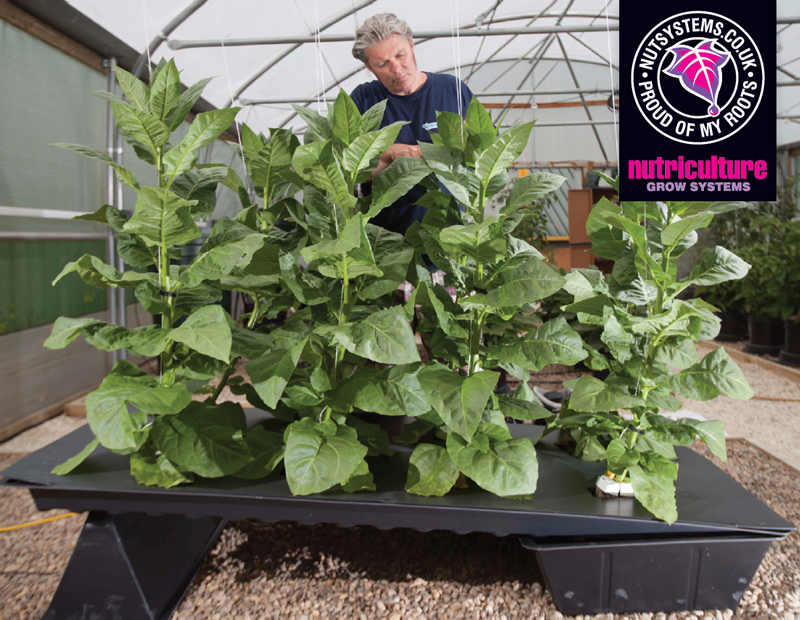The image depicts a man with grey hair, wearing a blue shirt, tending to tall, herbaceous plants with wide leaves inside a greenhouse. The plants are growing in a dark gray tray on a slightly tilted platform, supported by white strings attached to the ceiling. The man seems to be concentrating on his task. On the top right corner of the photograph, there's a circular logo containing a purple and pink leaf with a droplet, along with the text "nutsystems.co.uk" at the top and "proud of my roots" at the bottom. Beneath the emblem, the words "NutriCulture grow systems" are displayed, with "NutriCulture" in pink and "grow systems" in pale purple. A black rectangular box with the same text and logo is also visible in the background of the greenhouse, suggesting that the image might be promoting a plant growth system. Rocks are visible below the platform, adding to the greenhouse setting's realistic detail.